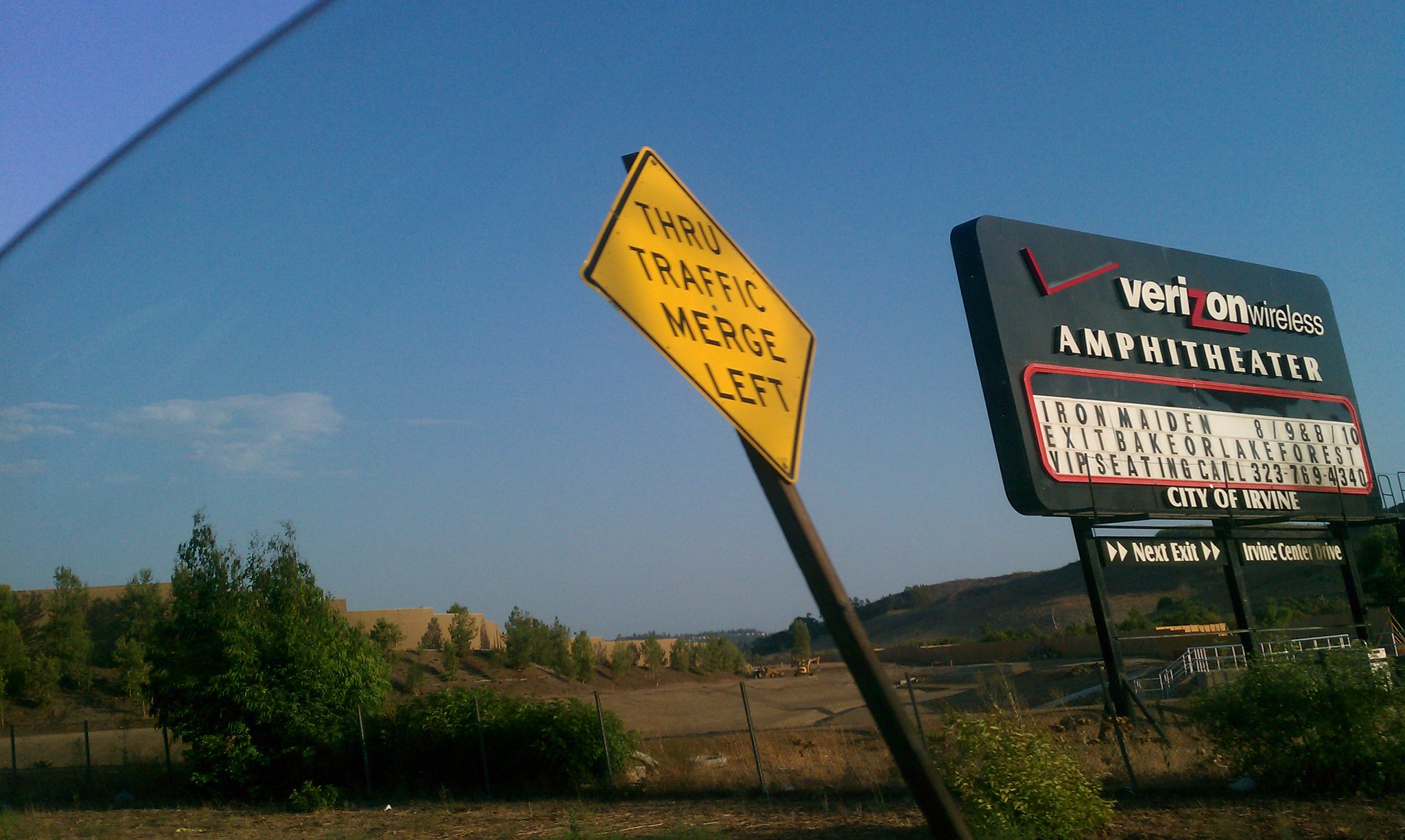The image, likely captured from the passenger side of a vehicle, offers a detailed roadside scene. A prominent yellow diamond-shaped traffic sign with a black border indicating "Through Traffic Merge Left" is seen leaning backward at approximately a 40-degree angle. Nearby, a billboard for the Verizon Wireless Amphitheater in the City of Irvine also appears to be leaning backward, a visual effect caused by the wide-angle lens used to take the photograph. The billboard highlights upcoming performances by Iron Maiden and provides phone numbers for reservations or tickets.

In the background, a field or construction area is visible, bordered by a range of hills on the right side. Atop the left hill, several buildings constructed from tan-colored bricks can be observed. The immediate foreground is dominated by a large chain-link fence running across the image, further emphasizing the roadside setting.